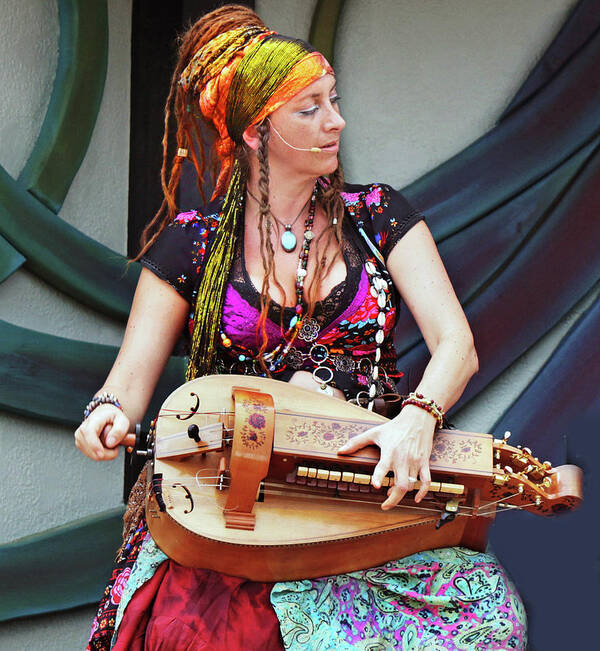This color photograph, in portrait orientation, features a Caucasian woman seated and playing a unique musical instrument on her lap. The backdrop consists of green and blue swirly loops against a white or beige background. The woman’s vibrant attire includes a multicolored, abstract-patterned short-sleeved dress with flowers and solids, and a scoop neck. She wears a colorful vest over a black lace shirt and a multicolored wrap skirt.

Her head is turned to the right with eyes lowered, showcasing a colorful head wrap in shades of lime green, orange, yellow, and gold, adorned with beads and braids. Brown bead-braided hair extends from both sides of her face, with additional braided extensions piled on top and cascading out from the back like a ponytail.

She is equipped with a small headset microphone that extends from her ear to her mouth. Around her neck, she wears a turquoise necklace. The instrument she holds is ornate and resembles a hurdy-gurdy with keys to play notes, a short fretboard, and a crank she turns with her right hand. The overall aesthetic appears to blend photographic realism with representationalism, capturing the intricate details and rich colors vividly.